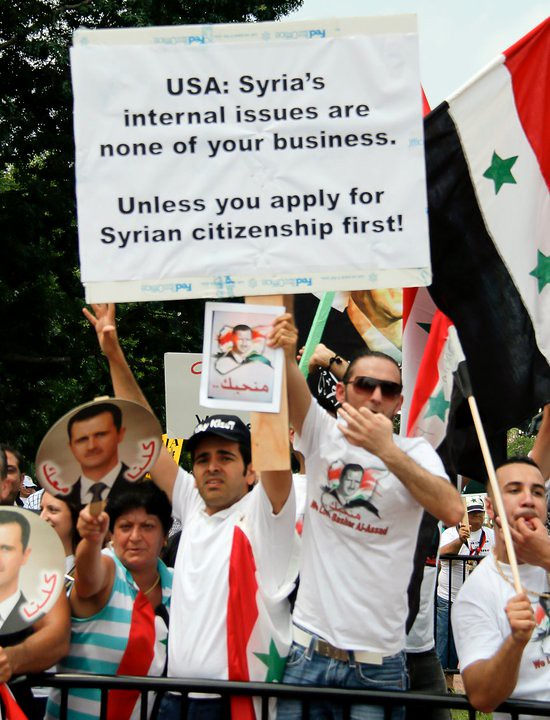A photograph captures a spirited Syrian protest, with around a dozen demonstrators standing behind a black guardrail. The protesters are holding a variety of signs and a Syrian flag. One prominent sign reads, "USA: Syria's internal issues are none of your business unless you apply for Syrian citizenship first." The Syrian flag, featuring a red top stripe, a white middle stripe with two green stars, and a black bottom stripe, is held up in the top right corner of the image. The protesters are dressed mostly in short-sleeved shirts, indicating a warm, likely summer day. Among them, some wear shirts adorned with a person's face, possibly the Syrian president, which appears to be a common theme in their signs and hand-held paddles. The background is dotted with green trees, adding a touch of nature to the scene. One protester at the bottom right corner is captured mid-action, seemingly about to whistle, contributing to the energetic atmosphere. The overall setting reflects a passionate assembly of Syrian nationals advocating for their cause.